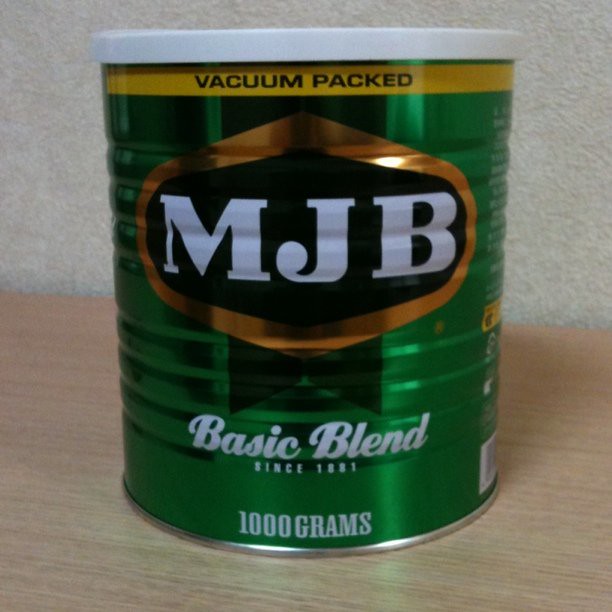This image features a green canister with a white top and a prominent golden banner underneath the lid, which reads "Vacuum Pact." Centrally displayed on the canister is the product logo: "MJB" in bold white text set against a black spade with a golden outline. The inscription "Basic Blend since 1881" is also visible on the canister, along with the weight specification "1,000 grams." The canister is placed on a lightly colored wooden table.